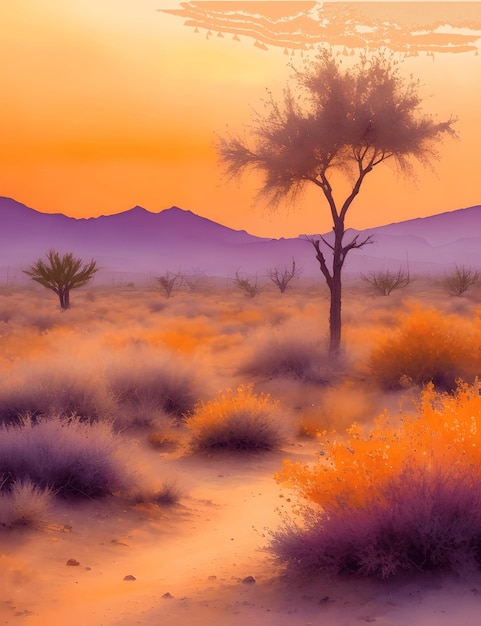This digital painting vividly depicts a desert landscape at sunset. The sky transitions from dark orange on the left to a lighter orange and yellow hue towards the right, with patches and dots of orange creating a striking horizon. Shadows in the top right corner give a sense of depth. In the distant background, purple mountains stand out against the vibrant sky. The foreground is populated with an array of desert vegetation, including purplish-gray and orange scrub and cactuses. A thin, bare tree with a bushy tan top stands prominently in the center, extending upwards. The ground is a mix of sandy dirt and scattered bushes, some green and others in shades of orange and brown. A meandering dirt path cuts through the base of the image. The overall scene captures the stark beauty and vivid colors typical of a desert at sunset, emphasizing the desolate yet strikingly beautiful environment.